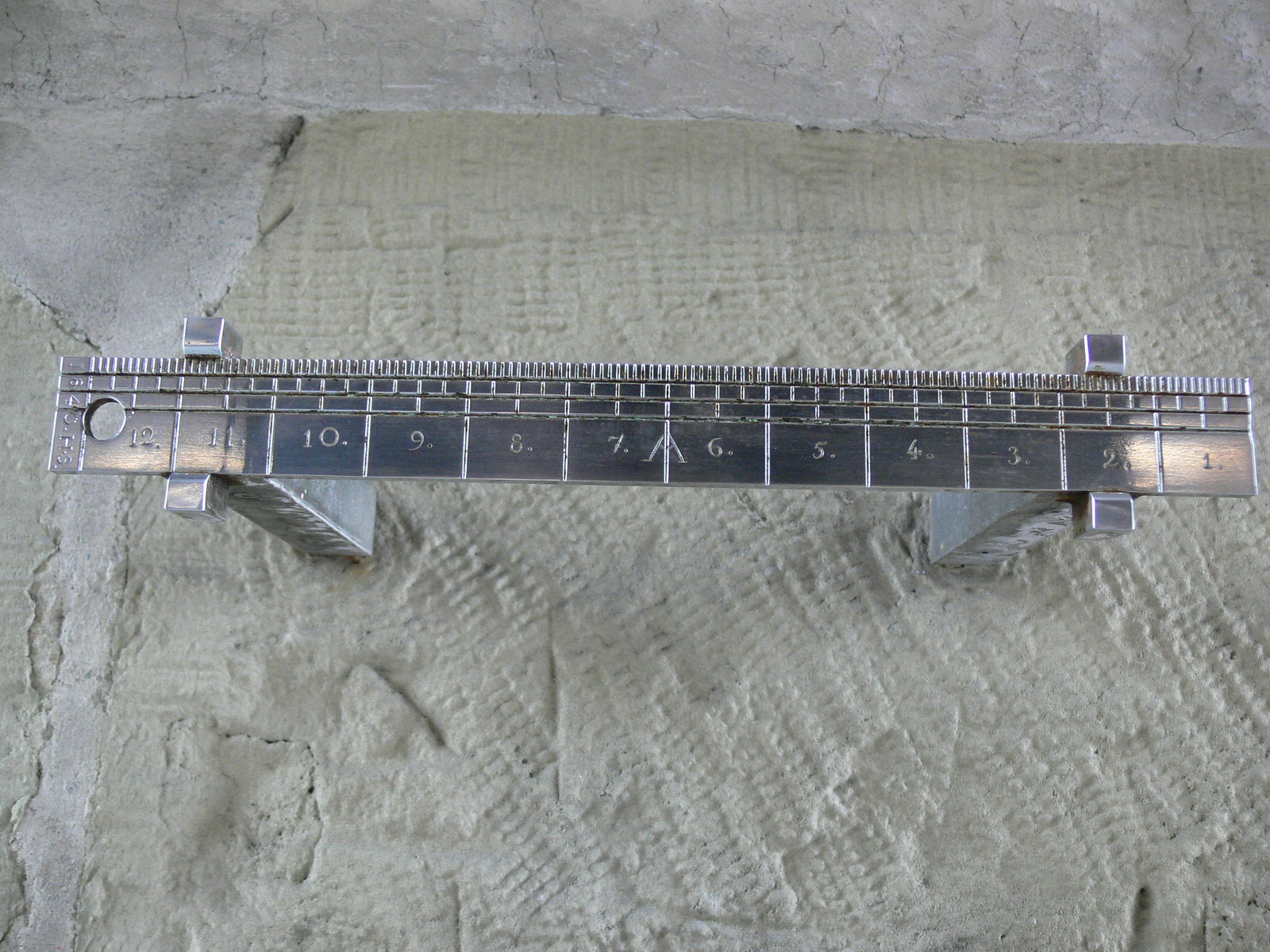This outdoor photograph features a metal ruler measuring device mounted atop two vertical metal posts set in what appears to be a textured, concrete floor. The concrete has distinctive marks, reminiscent of fork tines. The ruler, designed for precise measurements in woodworking, stonework, or similar projects, displays inch markings from 1 to 12, with subdivisions for half and quarter inches. A sliding calibration tool is situated at the bottom of the ruler for highly accurate measurements. Notably, there's a small hole on the left side of the ruler, and an arrow-like mark between the numbers 6 and 7. The surrounding backdrop includes a wall with a patch that appears freshly plastered, contributing to the overall industrious and functional setting of the scene.